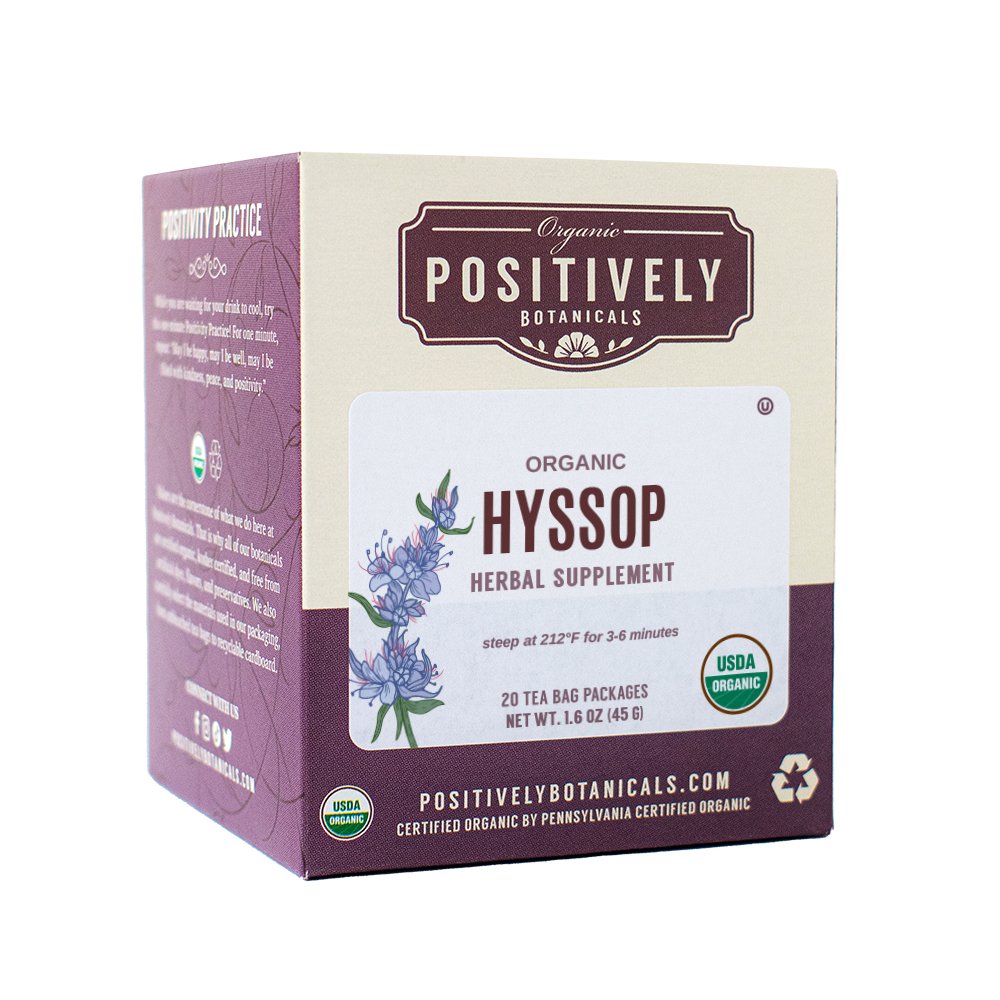The image depicts a box of Positively Botanicals Organic Hyssop Herbal Supplement, containing 20 tea bags with a net weight of 1.6 ounces (45 grams). The box is primarily in a light yellow or beige color with a dark red or plum-colored design, accented by white rounded rectangles that house the majority of the text. At the top, the logo "Organic Positively Botanicals" is prominently displayed in red letters, accompanied by a small flower illustration. The product is labeled as a USDA-certified organic supplement, with the USDA Organic logo appearing twice on the front of the box—once to the right under the main logo and again in the lower-left corner. Additionally, the label indicates that the product is certified organic by Pennsylvania Certified Organic. The front also instructs to steep the tea at 212 degrees Fahrenheit for three to six minutes. The bottom right corner displays a recycling symbol. A partially visible side of the box, dominated by the dark reddish color, seems to contain the company's mission statement, but it is out of focus. The image effectively showcases the supplement's packaging, emphasizing its organic certification and appealing design.